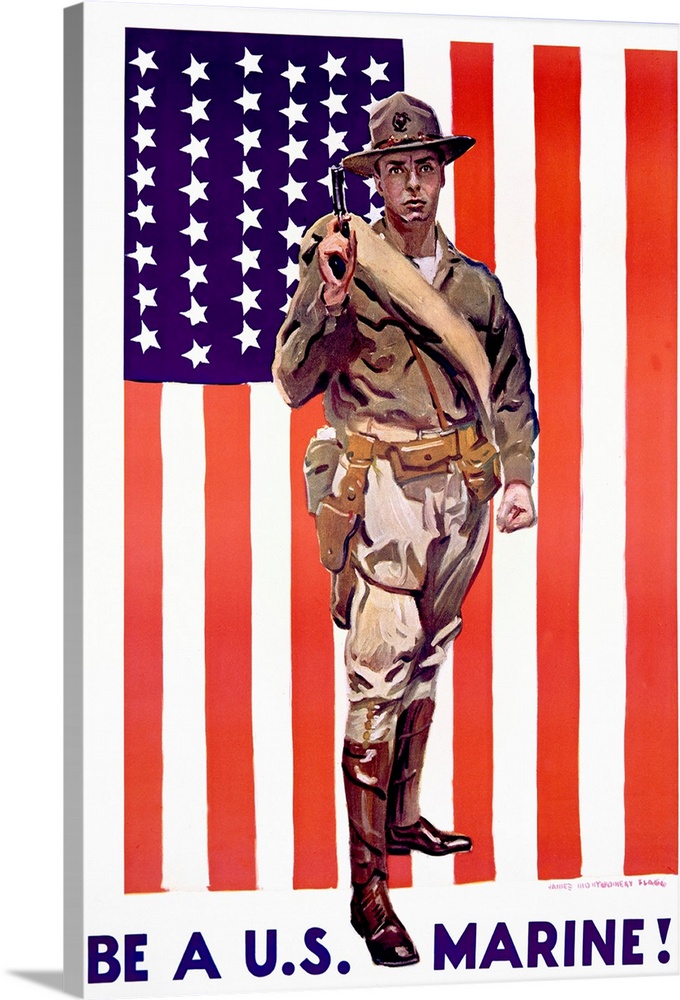The image depicts an old Marine recruitment poster set on a rectangular white frame, resembling a work of art potentially created with oil paint or some form of drawing. Dominating the background is the American flag, oriented vertically with the field of blue stars in the top left and red and white stripes running to the right and downward. Central to the image is a stern-faced enlisted Marine, dressed in traditional military attire which includes a tan jacket, tan or light gray trousers, and high brown boots. He dons a distinctive Marine Corps hat, described variably as a light gray hat or a white-brimmed cap, and a belt holster across his waist. His right hand grips a Colt 1911 automatic pistol, while his left hand is clenched into a fist. Draped around his chest is a structured scarf, adding to his resolute appearance. Below the main figure, bold blue lettering on a white background declares, "Be a U.S. Marine!" Though partially obscured, the artist’s name appears at the top of the poster. The overall aesthetic gives the poster a nostalgic, almost cartoonish feel, enhancing its vintage appeal.